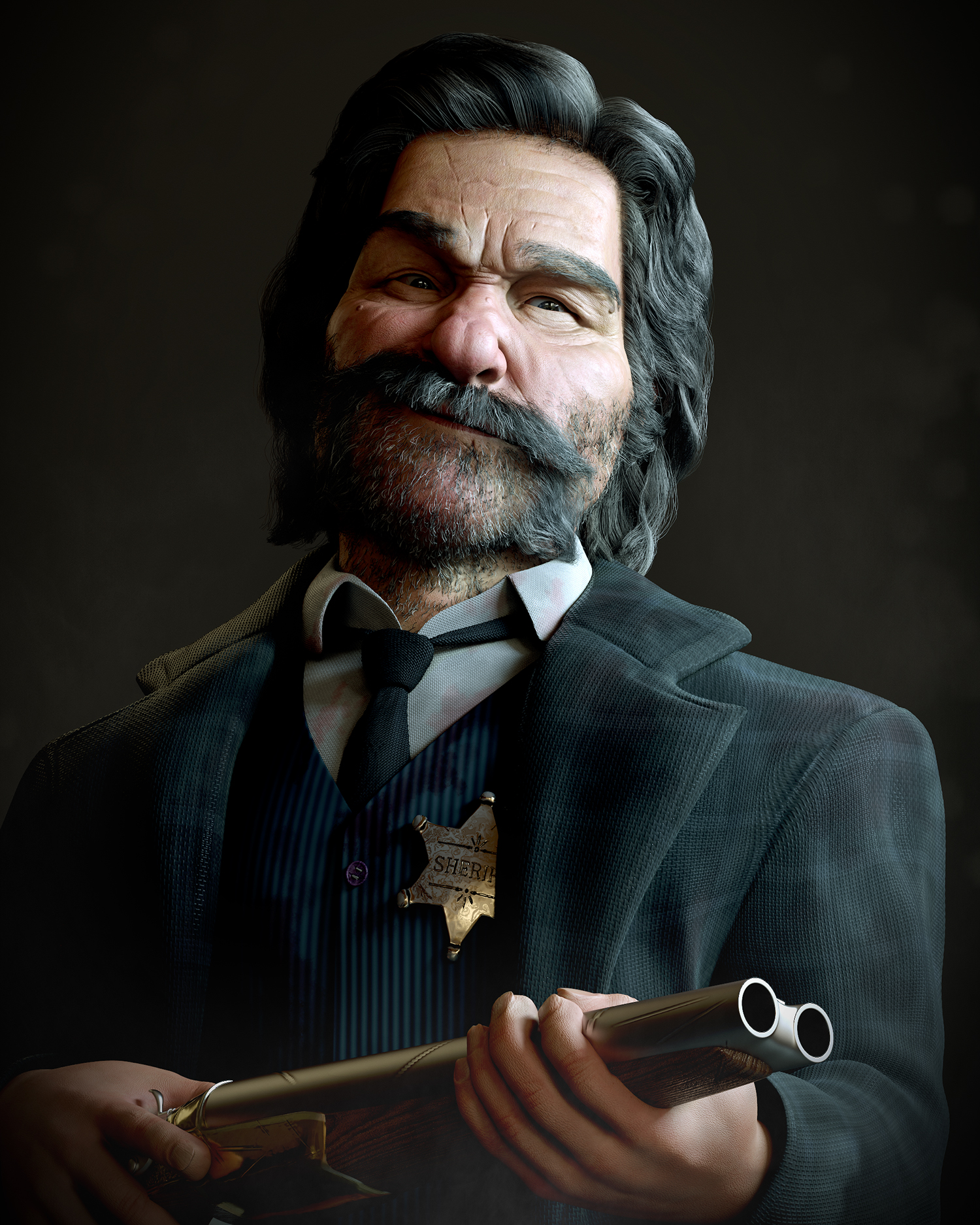The image features a highly realistic wax statue, possibly from a wax museum, depicting a man resembling a Sheriff from the 1800s. The statue has longish, salt-and-pepper hair reaching his neck, with thick, graying eyebrows and a distinct mustache that extends down the sides of his mouth. His chin also has hair, but it's sparser than the mustache. He wears a white shirt, a black tie, and a gray suit jacket over a vest adorned with green and black vertical stripes. A gold, star-shaped badge labeled "Sheriff" is prominently displayed on the left side of his chest. The man’s head is slightly cocked to his left (the viewer’s right). In his hands, he holds an old western-style, double-barrel shotgun, with his left hand near the barrel’s end and his right hand at the trigger. The background of the image is dark, accentuating the detailed and lifelike qualities of the statue.